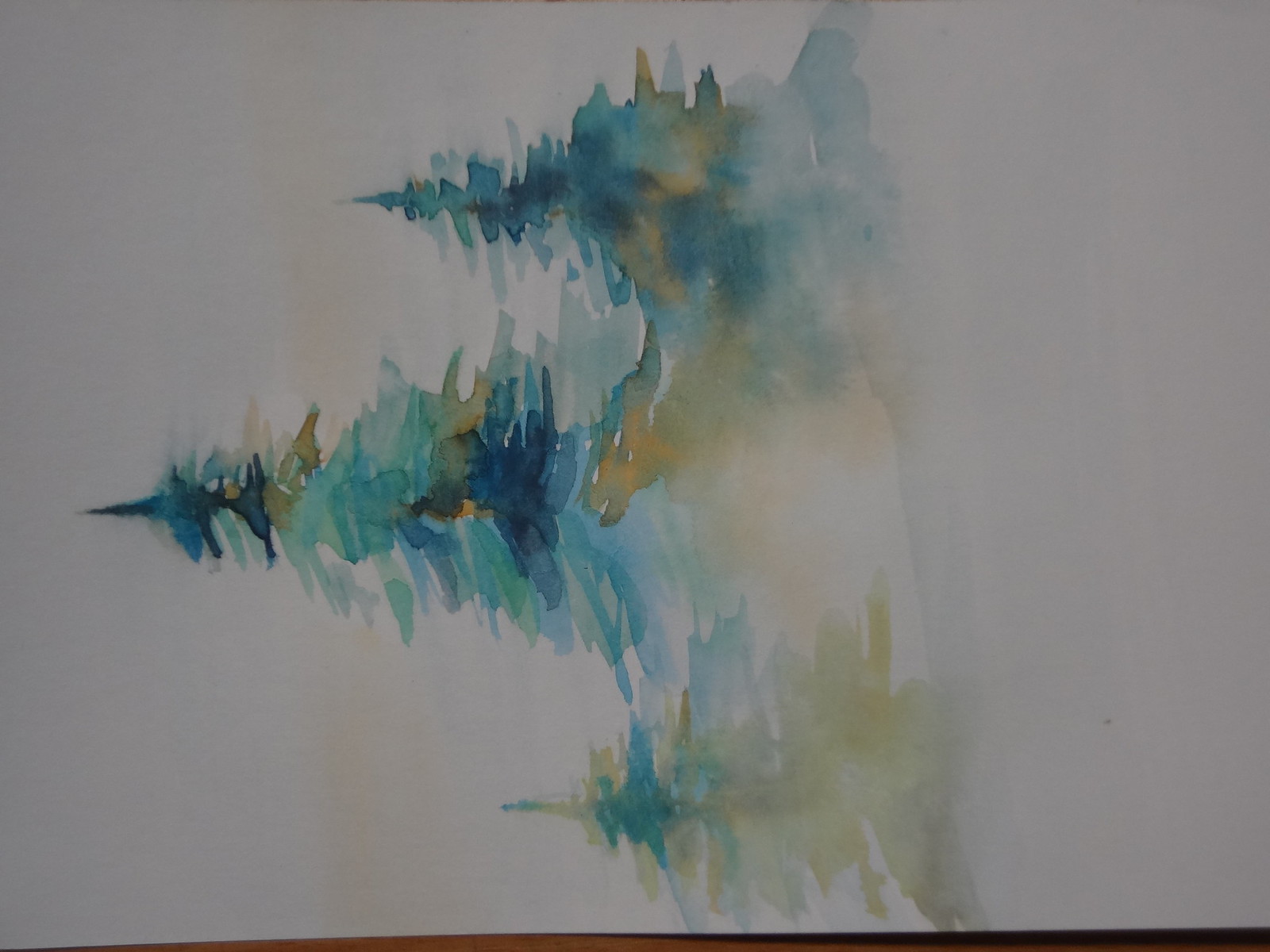The photograph captures a watercolor painting, notably rotated 90 degrees to the left, positioned on a flat, wooden brown surface. The painting itself showcases a bluish landscape, suggesting a snowy scape. Dominating the composition are three pine trees, rendered with various shades of blue, green, and yellow, creating a textured, triangular appearance. The tallest tree stands prominently in the middle, flanked by two smaller ones on either side. The background features an orangish-yellow skyline, enhancing the overall tranquility of the scene. The watercolor technique presents detailed tree tops that dissipate towards the bottom, melding into the indistinct landscape, giving an impressionistic touch to the evocative winter scenery.